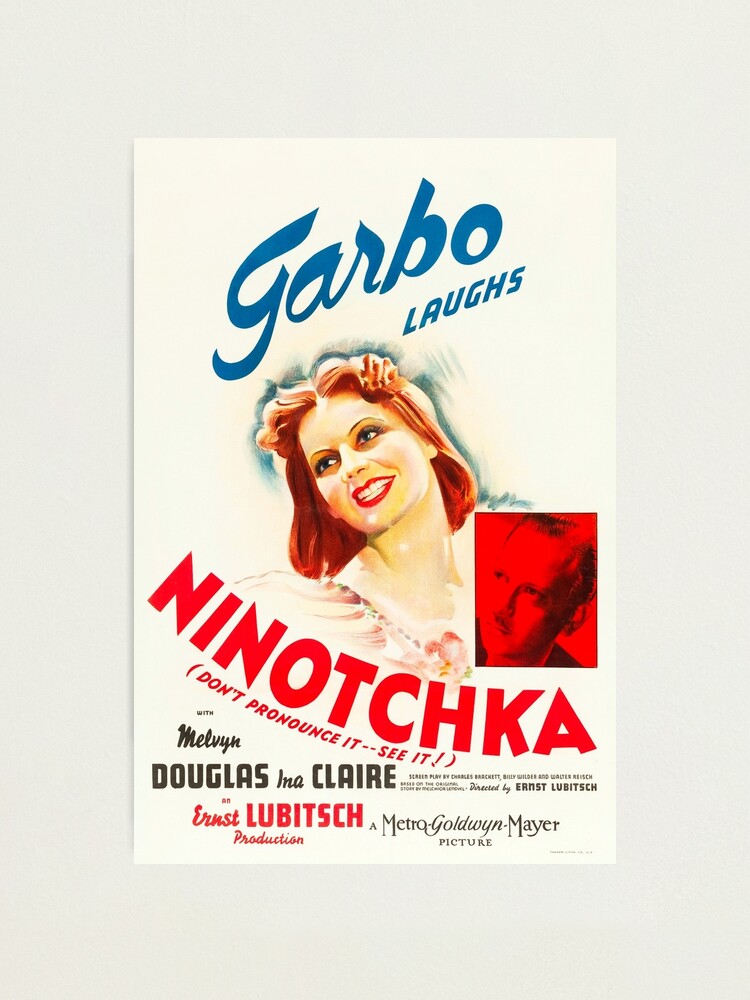The image depicts an old-fashioned movie poster with a light cream background. At the top of the poster, in dark blue font, are the words "Garbo Laughs." Below this, there is an illustration of a smiling woman with red hair styled fancily, adorned with blue eyes, and bright red lipstick. This image of the woman shows her from the shoulders up and she is tilting her head slightly. Below the woman's illustration is large red text that reads "Ninotchka." Underneath this, in smaller red font, it states, "Don't pronounce it - see it." To the bottom left of the poster, red text lists "Melvin Douglas, Ina Clare," followed by "an Ernst Lubitsch production, screenplay by Charles Brackett, Billy Wilder, and Walter Reisch," although the smaller text is somewhat difficult to read. Finally, on the right side of this information, it notes "a Metro-Goldwyn-Mayer picture." The overall design features a monochrome photograph of a man in red positioned to the lower right of the woman's illustration.